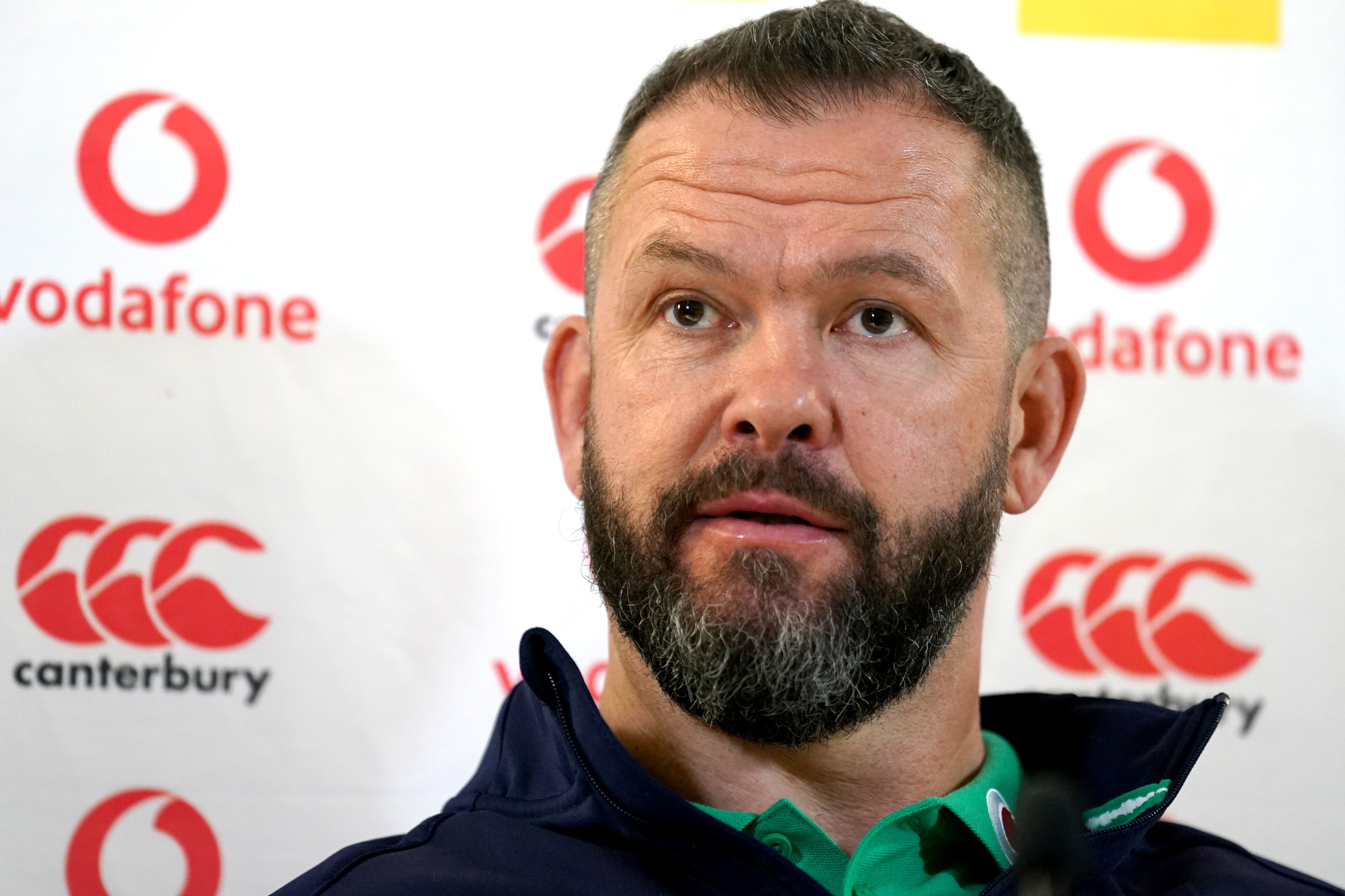The image depicts a close-up of a man standing in front of a white background adorned with two alternating company logos: one for Vodafone, featuring the word "Vodafone" in red lowercase letters beneath a red circular symbol, and another for Canterbury, displaying three overlapping red circles with a white bird silhouette and the word "Canterbury" in black underneath. The man, a white male with short black hair shaved close to the skull on the sides and thinning at the front, has a beard and mustache with noticeable gray streaks, particularly on the chin. He is wearing a blue jacket with a green pin and a black string, over a green button-down shirt with the first button open. The shirt has a red button on the right side of the collar. He appears to be looking slightly to the left, possibly engaged in conversation or at an event where he is being photographed.